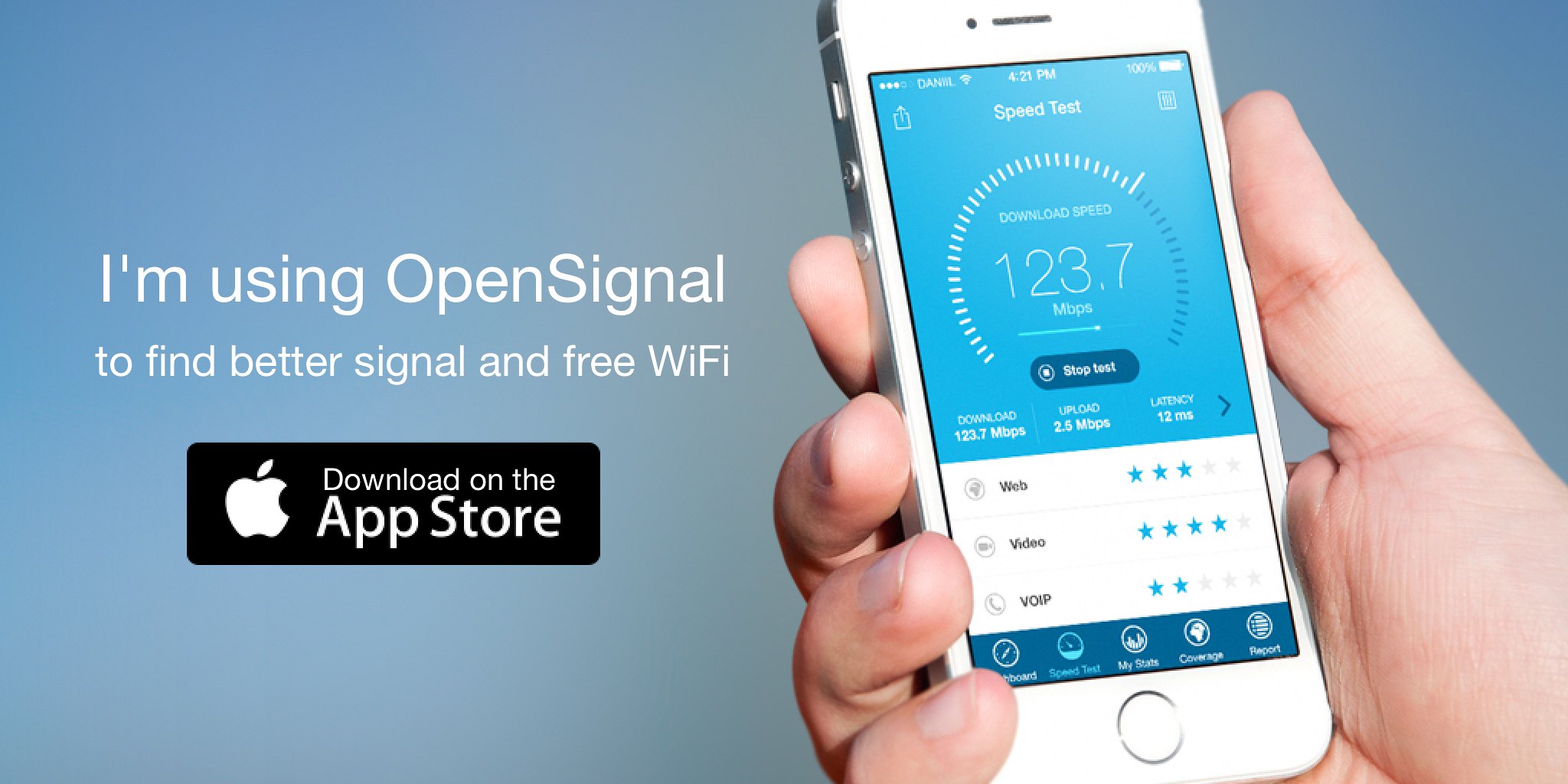The advertisement showcases an app available on the Apple Store called OpenSignal, set against a background with shades of blue. On the right side, a man’s hand is seen holding an iPhone displaying the app's interface. The screen prominently shows a speed test result with a download speed of 123.7 megabytes per second, along with other metrics listed below such as upload speed (2.5 Mbps), latency (12ms), web, video, and VOIP. To the left of the phone, the text reads, "I'm using OpenSignal to find better signal and free Wi-Fi." Below this, a black rectangle features the text "Download on the App Store" in white, accompanied by the Apple logo.